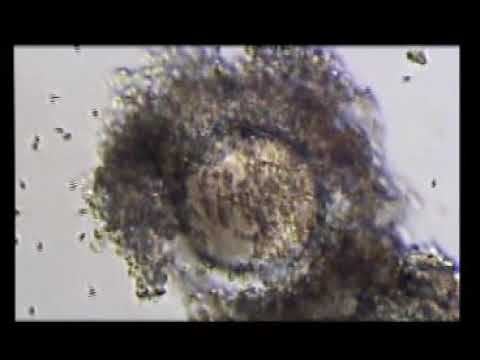This somewhat low-resolution image, framed by a black border, features a central circular area densely covered with what appear to be brown flies or granules. These elements give the impression of a biological or natural scene, potentially resembling a beehive or a microscopic view of bacteria. The flies or particles predominantly cover a head-like protective uniform or safety equipment, which is otherwise yellow in uncovered parts. Some of these flies are seen flying in the air against a light gray background, adding a dynamic element to the scene. The central object, detailed with brown and yellow hues amidst a predominantly gray and black palette, is surrounded by scattered bits and pieces, enhancing the intricate and somewhat ambiguous nature of the image.